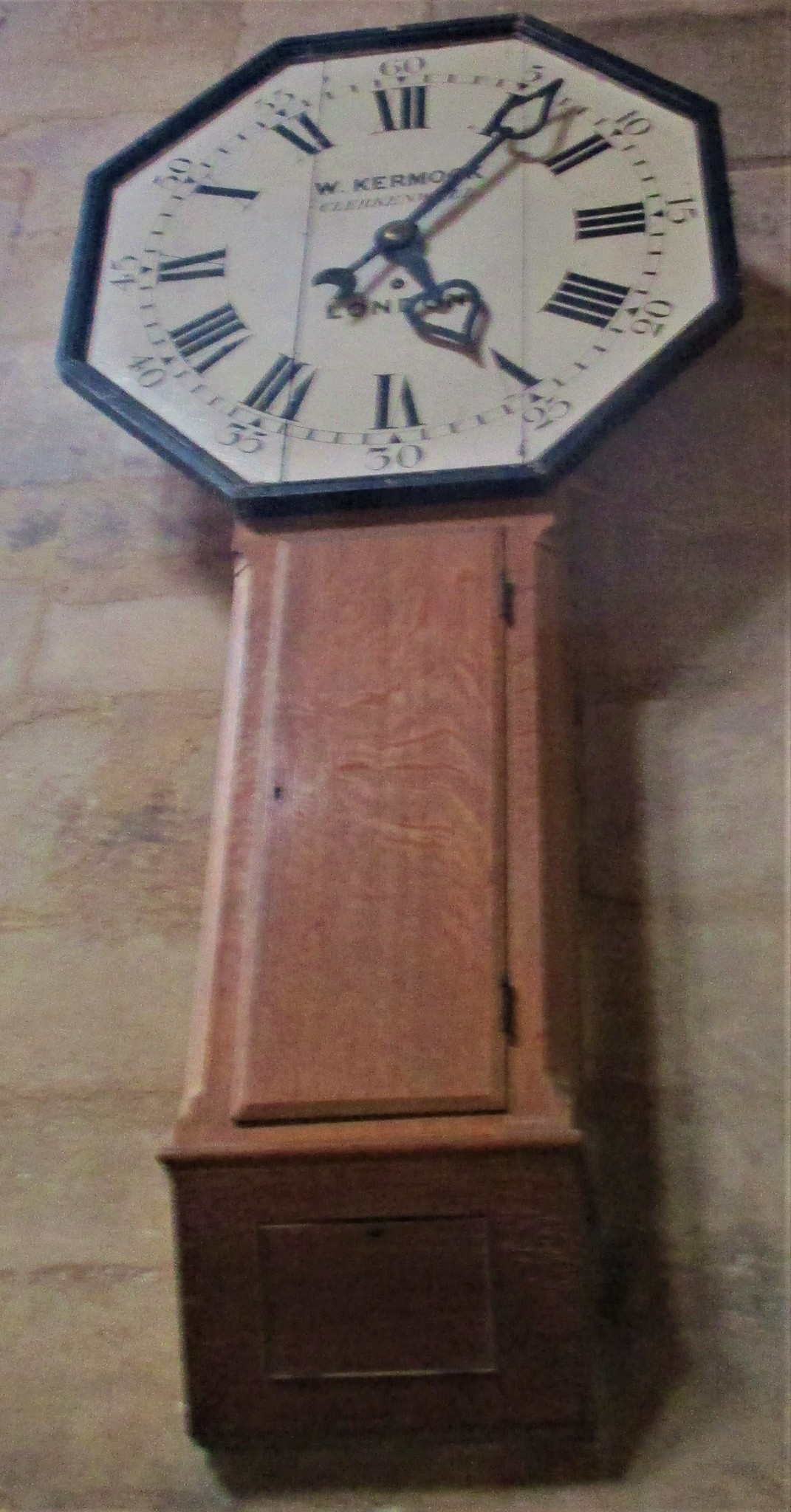The image features a wall-mounted clock captured from a low-angle perspective, creating an upward view. At the top of the photograph is the clock's face, encased in an octagonal frame. The clock's face is white, providing a stark contrast to the dark, elongated wooden base that extends downward. The hands of the clock indicate the time as 5:07. The unique composition of the picture highlights both the underside and the front of the clock, emphasizing its design and structure.